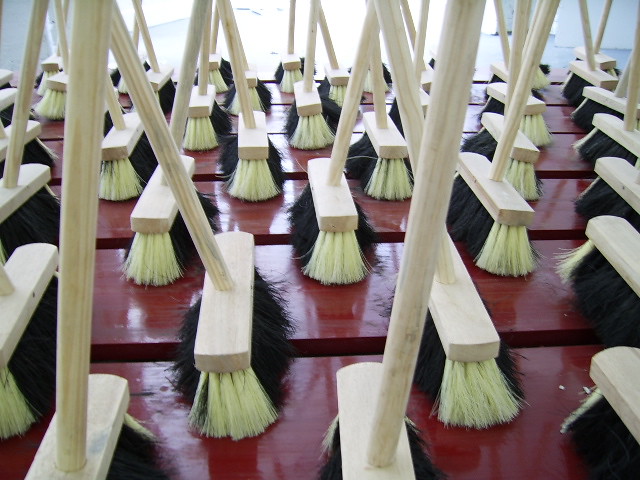This photograph features an array of approximately 30 to 50 unusual broad push brooms, meticulously aligned in an upright position. Each broom is constructed with a wooden handle made from light-colored, seemingly unfinished wood, giving it a raw, sanded-down appearance. The bristles of these brooms are distinctive, with the central bristles being black and the outer bristles fading to a blonde or light yellow hue, reminiscent of a skunk's coloration. These bristles are further secured by a wooden bar, likely a 2x4, which shares the same light wooden look as the handles. The brooms are neatly positioned atop broad, dark red wooden slats or planks, with a notable shine and some reflections visible across their surface. Despite the brooms' regimented arrangement, there is an intriguing interplay of light and shadow, enhancing the scene with additional depth and dimension. Though the top ends of the broom handles are not visible, they are likely held in place by an unseen support. The setting and details create a visually compelling and orderly presentation of these practical tools.